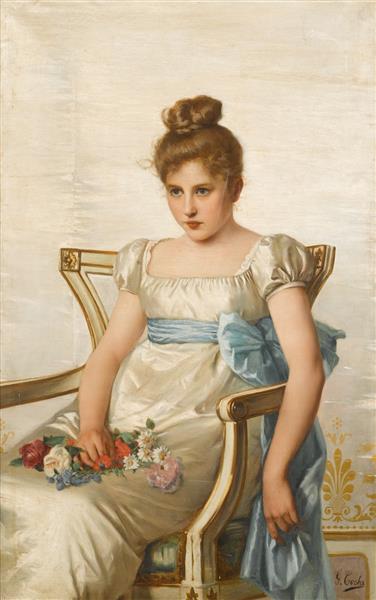This highly realistic oil painting features a young girl, likely around 12 or 13 years old, with fair skin and brown hair neatly tied up in a bun. She sits slightly slumped over in a large chair, which has a white frame with gold painted outlines, with the perspective capturing her from a side quarter angle on the left. Her gaze is directed forward.

The girl is dressed in a cream-colored satin dress with short, puffy sleeves. The fabric's shine is beautifully captured through the artist’s use of folds and highlights. Around her upper waist, just below her bosom, is a thick, sky-blue bow tied into a large sash that drapes prominently on her left side. In her lap, she cradles a small bouquet of daisies and other flowers, holding them with her right hand while her left hand rests on the bow's ribbon. 

The background is a beige white color, adorned with a subtle yellow fleur-de-lis design on the bottom right. The artist’s signature is also present in this area but is not legible. The painting stands out for its soft yet highly detailed and realistic depiction.